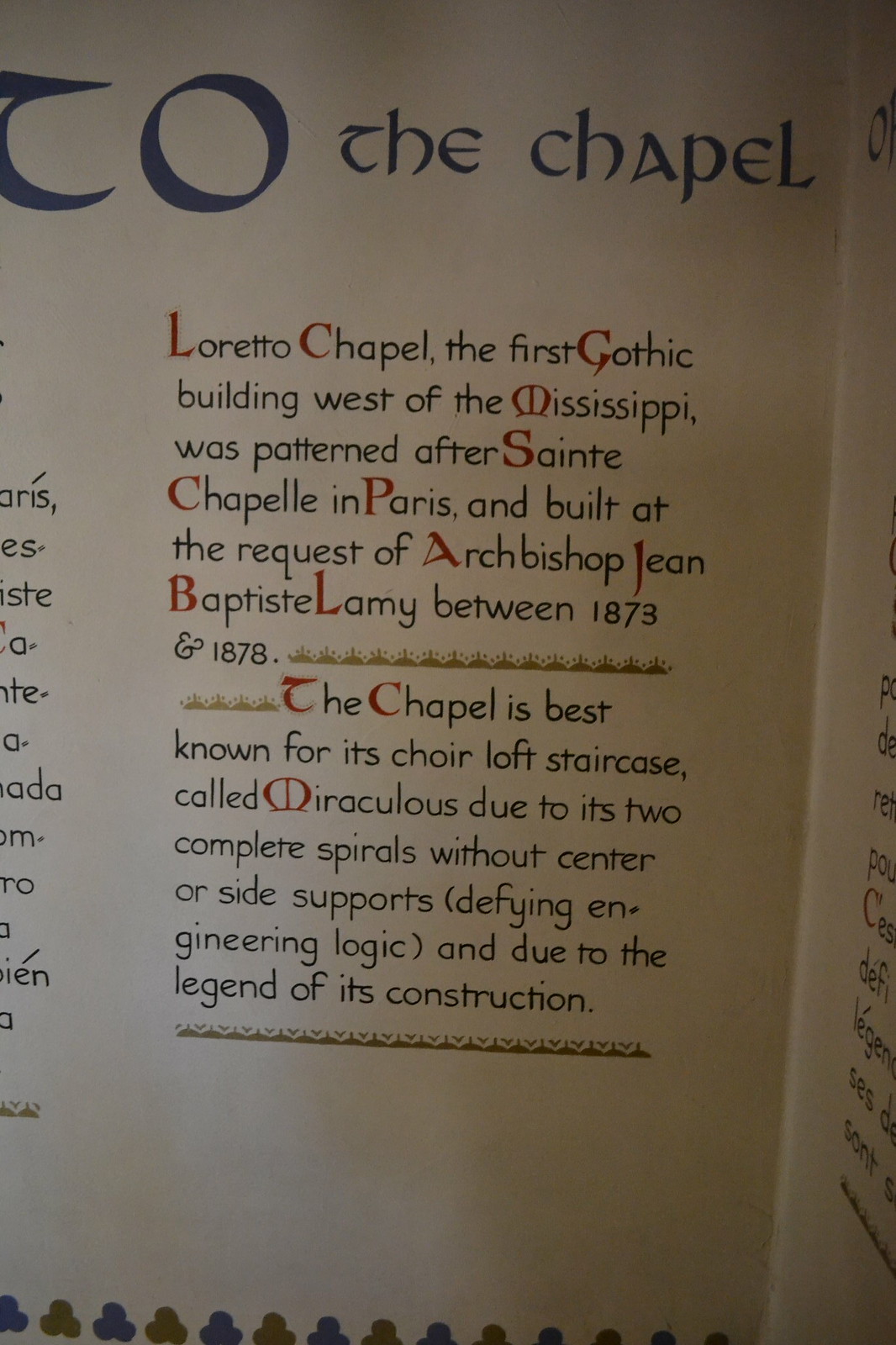The image depicts a photograph of a sign or page from a historical booklet, possibly related to the Loretto Chapel. The photograph is of a tall, rectangular page with medieval-looking blue text at the top, stating "To the Chapel." The main text beneath is printed in a black, old-timey font with occasional bright red capitalized letters. This text reads, "Loretto Chapel, the first Gothic building west of the Mississippi, was patterned after Sainte-Chapelle in Paris and built at the request of Archbishop Jean-Baptiste Lamy between 1873 and 1878. The chapel is best known for its choir loft staircase, called miraculous due to its two complete spirals without center or side supports, defying engineering logic, and due to the legend of its construction." Visible in the photograph are decorative details, including a floral pattern made of three intersecting circles in blue and red at the bottom of the page. The page appears to be part of a book, as indicated by a vertical crease starting from the top right corner and widening as it goes down. The background wall is off-white, intersecting with another wall on the right side, adding a contextual backdrop to the image.